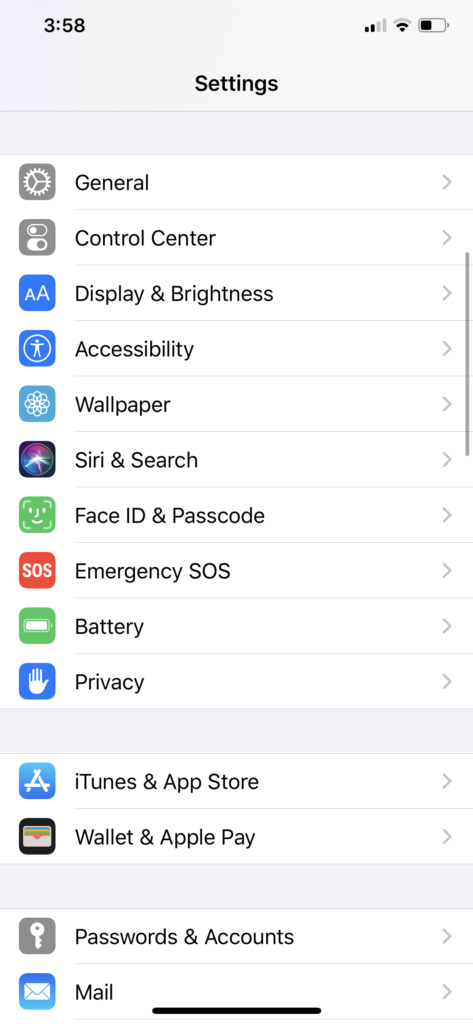The image displays a smartphone screen with the settings application open, showcasing various configuration options. At the top left corner, the time is indicated as 3:58, while the top right corner features several status icons, including battery level, Wi-Fi signal, and cellular signal strength.

The settings menu lists multiple options, each accompanied by distinct icons:
1. **General**: A grey and white gear icon.
2. **Control Center**: A grey and white toggle switches icon.
3. **Display & Brightness**: A blue icon with two white 'A's.
4. **Accessibility**: A blue icon featuring a person.
5. **Wallpaper**: A light blue and white image icon.
6. **Siri & Search**: A black and blue icon with purple, green, and red colors representing Siri.
7. **Face ID & Passcode**: A green icon with a white outline of a face.
8. **Emergency SOS**: A red icon with "SOS" written in white.
9. **Battery**: A green icon with a white battery symbol.
10. **Privacy**: A blue icon with a white hand symbol.
11. **iTunes & App Store**: A blue icon with the iTunes logo.
12. **Wallet & Apple Pay**: A black icon depicting a wallet.
13. **Passwords & Accounts**: A grey icon with a key symbol.
14. **Mail**: A blue icon with an envelope symbol.

Each option is arranged in a neat, vertical list format, allowing users to navigate to more specific settings by selecting any of the listed items.